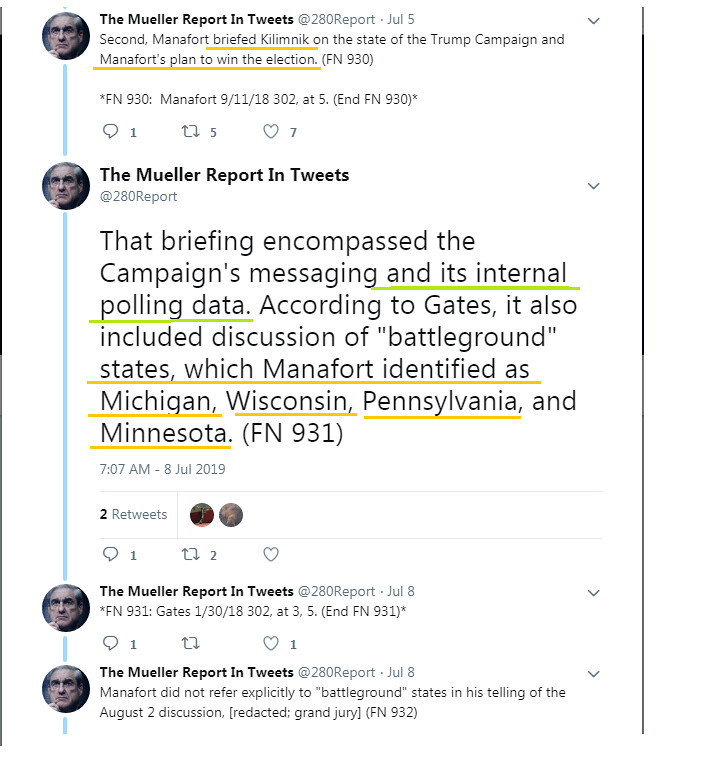This image features a compilation of tweets from the Mueller report, focusing on Paul Manafort and the Trump campaign. At the top of the image, there is a small circular profile picture of Robert Mueller, in black and white, accompanied by the text "The Mueller Report in Tweets." The main tweet details that on July 5th, Manafort briefed Kilimnik on the state of the Trump campaign and his strategies to win the election, with a parenthetical reference to FN 930. It continues, noting the briefing included discussions of campaign messaging, internal polling data, and battleground states such as Michigan, Wisconsin, Pennsylvania, and Minnesota, sourced from Gates, and referenced as FN 931 dated 7:07 AM, July 8, 2019. Below these tweets, additional entries consistently labeled "The Mueller Report in Tweets" are present, although their content is less detailed. This image also features typical Twitter engagement icons— a cloud (for replies) showing counts, an up and down arrow (for retweets) with counts, and a heart (for likes) with counts. The repetitive inclusion of "The Mueller Report in Tweets" emphasizes the ongoing, detailed updates provided in this format.